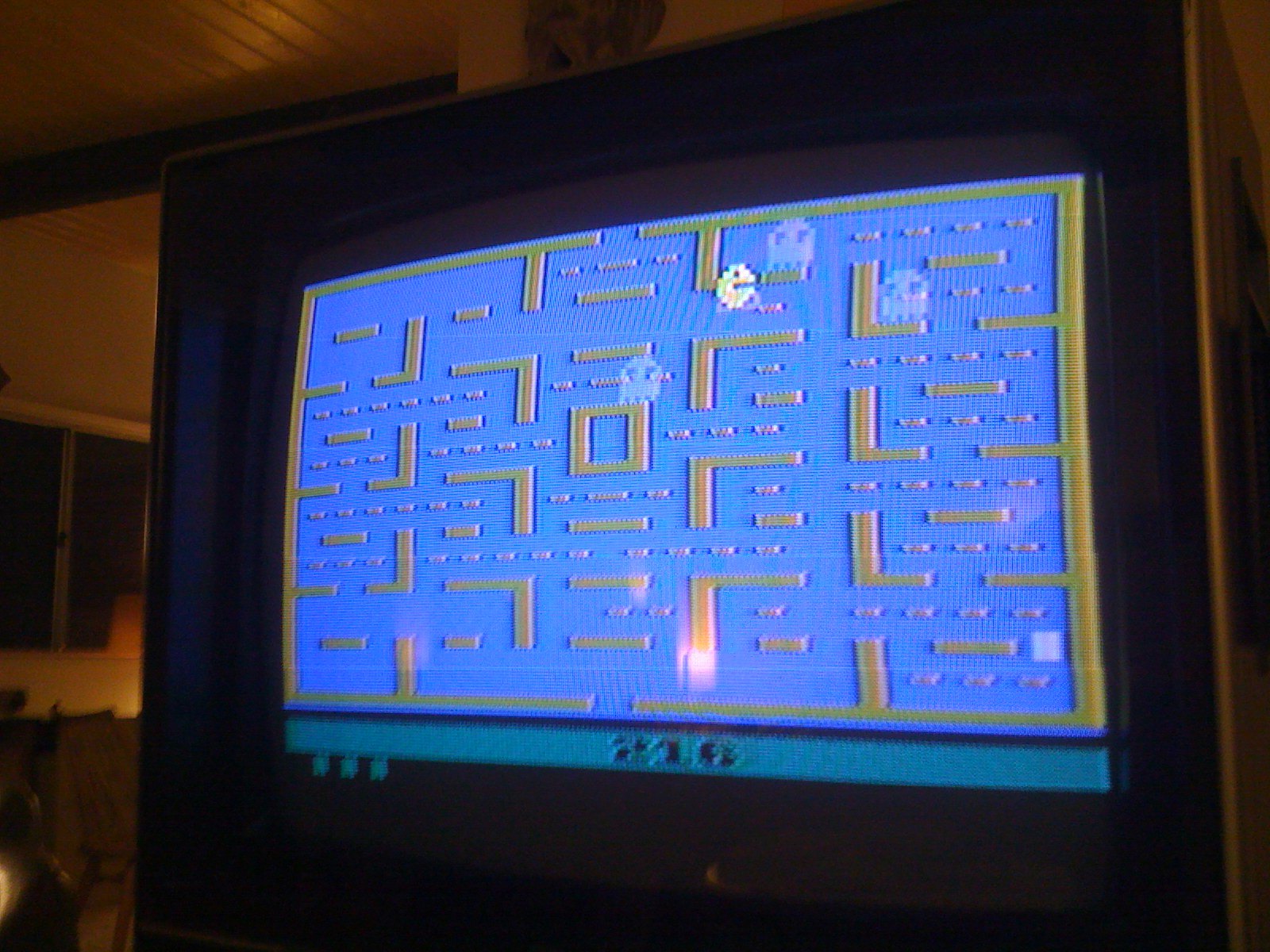This vintage photograph captures a cozy living room setting, centered around a classic home television encased in a wood-paneled cabinet. The TV screen, bordered by a substantial black frame, displays a game of Pac-Man in progress. The rudimentary graphics showcase a blue background with a brownish grid pattern typical of the era. On the screen, the iconic yellow Pac-Man character navigates the maze, pursued by three ghost figures, each with their distinctive colors. At the bottom of the screen, the score reads "216," indicating the player's current points, accompanied by a trio of dots and a white-green status bar. The ambient lighting softly illuminates the room, revealing a glimpse of the ceiling above and a dimly lit adjacent space with a window visible on the left side. This nostalgic image evokes a sense of retro gaming charm and homely comfort.